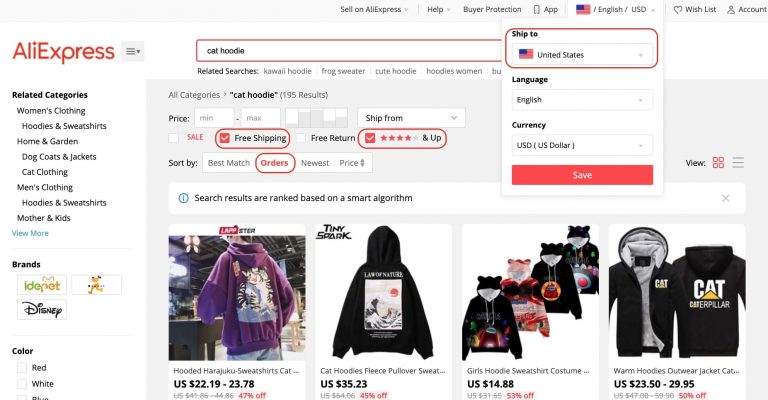The image is a screenshot of the AliExpress website, showcasing various features and categories. At the top left corner of the image, the AliExpress name is displayed in red. Adjacent to it on the right, there is a gray square containing a hamburger menu icon. Moving towards the top right, the word "Account" is visible, with other navigation options extending towards the left, including "Wishlist," "English," "USD," "App," "Buyer Protection," "Help," and "Sell on AliExpress."

On the far left side of the image, directly underneath the AliExpress title, several specific categories are listed under the bolded heading "Related Categories." These categories include "Women's Clothing," "Hoodies and Sweatshirts," "Home and Garden," "Dog Coats and Jackets," "Cat Clothing," "Men's Clothing," "Hoodies and Sweatshirts," and "Mothers and Kids." Below these categories, a "View More" link in light blue is present, leading to additional categories.

Further down, the word "Brands" is prominently shown, followed by three boxes depicting different brands. The top-left box is labeled "Ido Pet," the bottom box is marked "Disney," and the top-right box features an illustration of a yellow dog without any text.

In the center of the image, towards the top, there is a search bar with the input text "cat hoodie," indicating the current search query on the website.